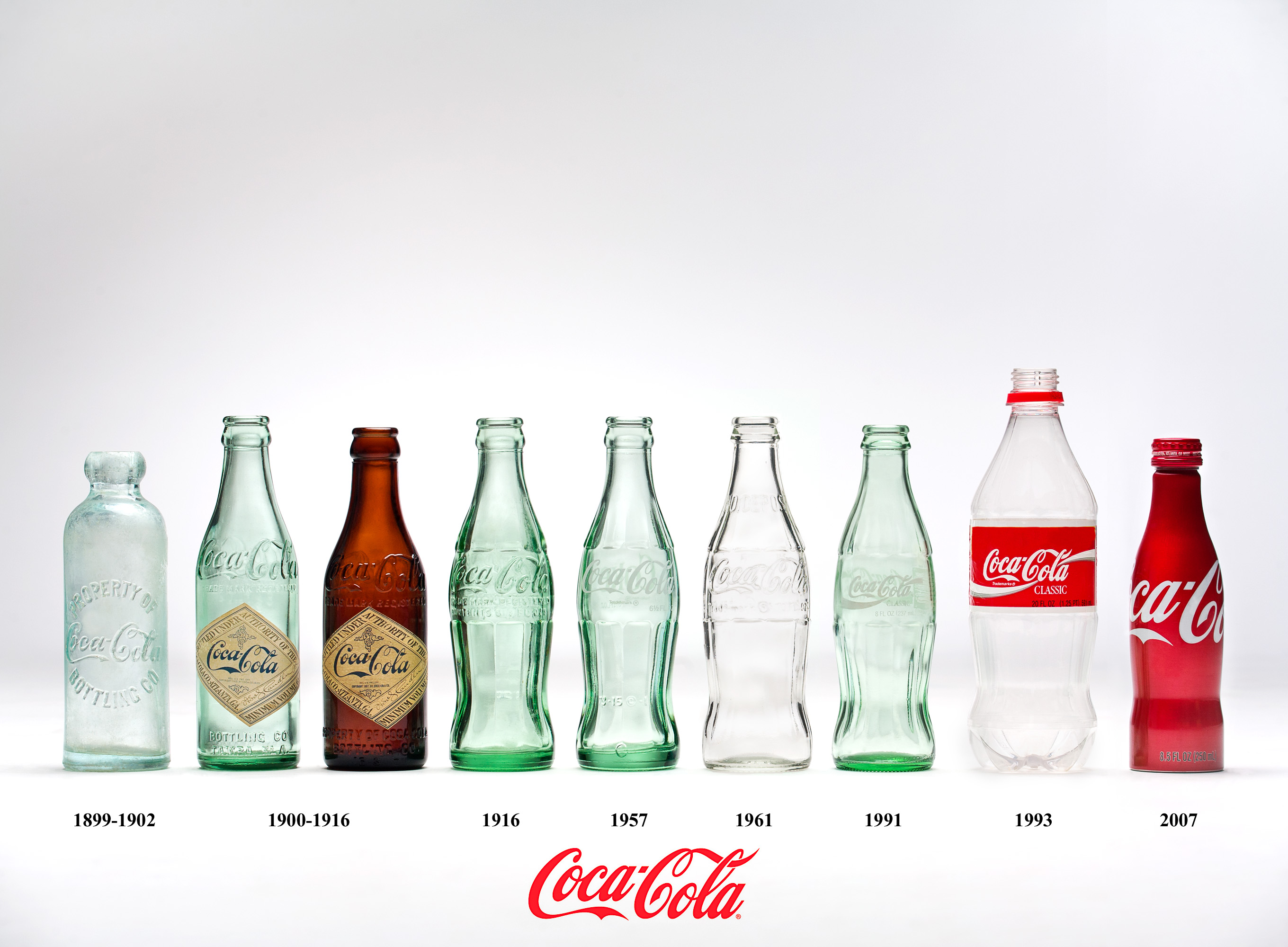The photograph showcases the evolution of Coca-Cola bottle designs in a timeline fashion. Against a pure gray background, the image features a line of nine different Coca-Cola bottles, each designated with a range or specific year beneath it in black print, and the iconic Coca-Cola logo at the bottom center. 

Starting from the left, the first bottle is from 1899 to 1902, which is a clear bottle with a slight bluish tinge and a very short neck, embossed with "Property of Coca-Cola Bottling Company." Next, spanning from 1900 to 1916, are two bottles: one with a greenish tint and a longer neck, the other amber-colored with raised print and light brown diamond-shaped stickers labeled "Coca-Cola."

Following these, we have the 1916 Coca-Cola bottle, which is taller, more green, and features a thin inverted band with raised "Coca-Cola" text. The 1957 bottle is similar but slightly lighter in green, while the 1961 bottle is clearer and whiter. The 1991 bottle is smaller and greener, both shorter and thinner than its predecessors.

The 1993 bottle marks the transition to plastic, featuring a red cap and a red banner with white "Coca-Cola Classic" print. Lastly, the 2007 bottle is made of aluminum, painted red with white "Coca-Cola" print, and beneath all bottles is the Coca-Cola logo in red cursive, set against the consistent gray background.